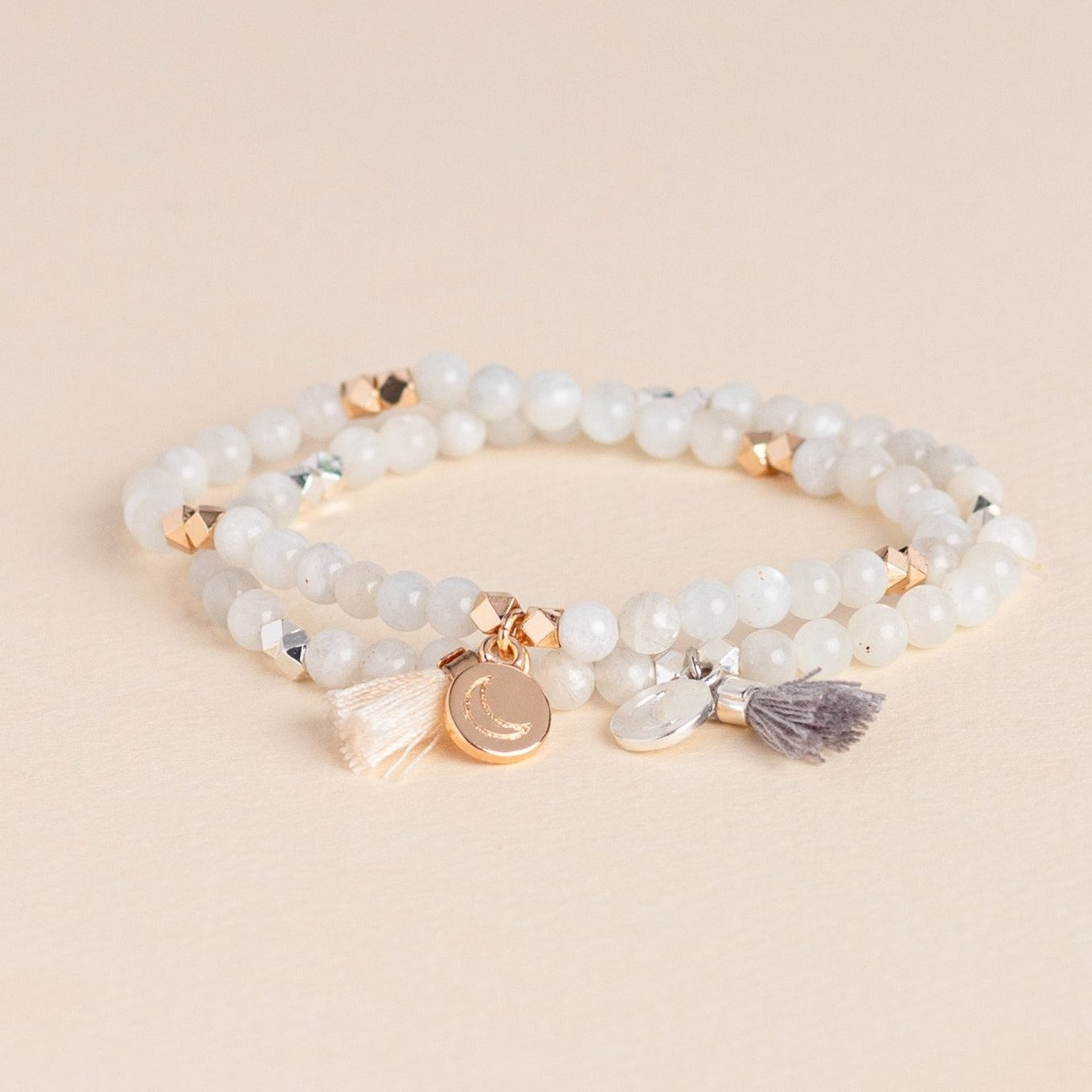The product image showcases two intricate, handmade beaded bracelets elegantly laid on a peach-colored background. The bracelet on top features lustrous pearl-colored beads separated by rose gold tetrahedron beads. Attached to it is a delicate cream-colored tassel and a small, round rose gold pendant engraved with a moon, adding a touch of celestial charm. Below it, the second bracelet consists of white pearl beads interspersed with silver divider beads. This bracelet includes a rich purple tassel and a matching round silver pendant, similarly engraved with a moon motif. The harmonious combination of pearls, rose gold, silver, and the soft hues of the tassels, against the peach backdrop, creates a visually captivating and detailed representation of these dainty yet sophisticated pieces of jewelry.